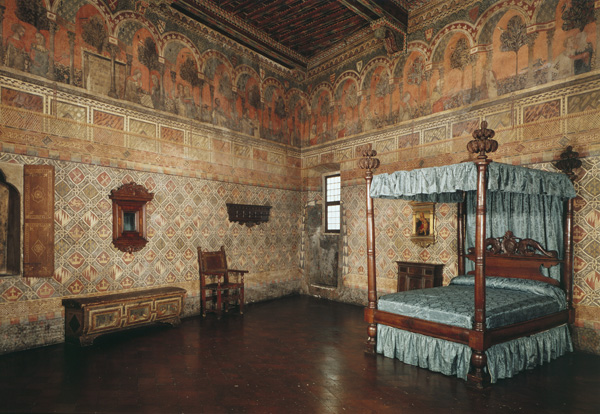This photograph captures a spacious, vintage bedroom with impressively high ceilings, possibly reaching up to 20 feet. The room's decor is reminiscent of late 1700s to 1800s European style, characterized by its ornate and somewhat gaudy aesthetic. Dominating one wall is a four-poster bed crafted from dark wood, with ornate carvings on the headboard and tops of the posts. The bed is adorned with a dusty blue silk canopy connecting all four posts, matching the light blue bedspread and ruffled bottom. Behind the headboard, a curtain of the same blue silk drapes elegantly.

The walls are covered in intricate, busy wallpaper that has faded with age. The wallpaper features an orange diamond pattern on a taupe background, with orange, cream, and brown arches at the top. The ceiling continues the room's vibrant theme with multicolored stripes. Despite its rich decorations, the wallpaper and overall color palette have dulled to various shades of beige, brown, and gray due to age.

Adding to the historical ambiance, the room includes wooden furnishings typical of old Europe, such as a finely crafted wooden chair. The floor is made of dark, shiny wood, adding a touch of elegance to the room. In the corner, near the middle of the image, a small window provides a hint of natural light, subtly illuminating the space.